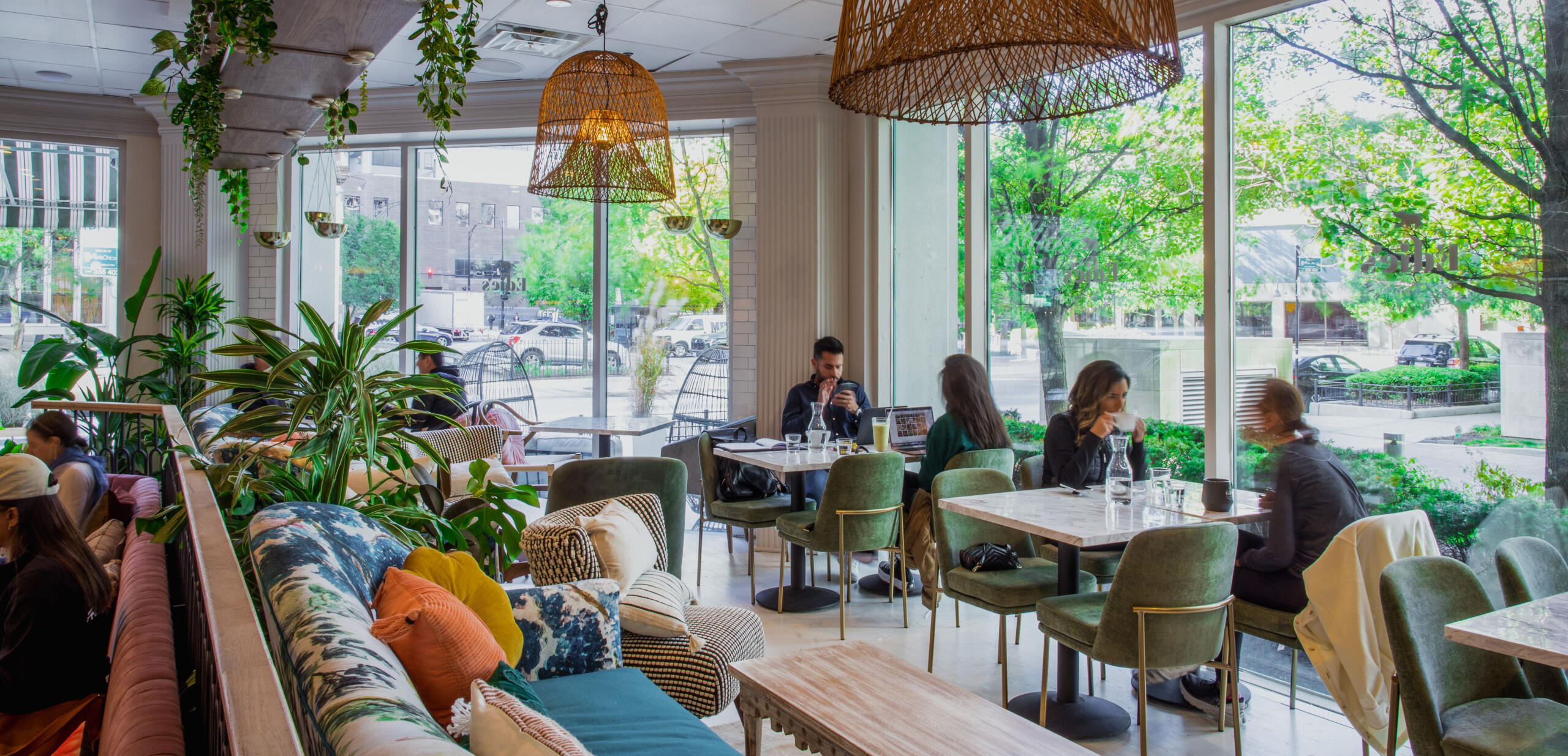The photo captures a chic, mid-tier boutique cafe, bathed in daylight streaming through large, transparent glass windows that offer a view of the vibrant street outside, lined with parked cars and lush green trees. Inside, the cafe boasts a stylish and eclectic interior design. To the left, a blue couch adorned with colorful throw pillows sits in front of a wooden table, providing a cozy nook for patrons. On the right, green chairs surround tables, where two couples sit face to face, enjoying their meals and engaging in lively conversations. Additional seating includes a mix of sofas and chairs, some occupied by people using laptops and engaging with one another.

The ambiance is accentuated by white ceilings with hanging basket-shaped chandeliers emitting a warm, yellow-orange glow. Vines and green indoor plants, such as ferns and Monsteras, add a touch of nature, cascading from the ceiling and settled throughout the space. The spread-out tables and comfortable seating arrangement create a welcoming atmosphere, perfect for a leisurely brunch. The setting exudes a balanced mix of modern and cozy, making it an inviting spot for both relaxation and socialization.